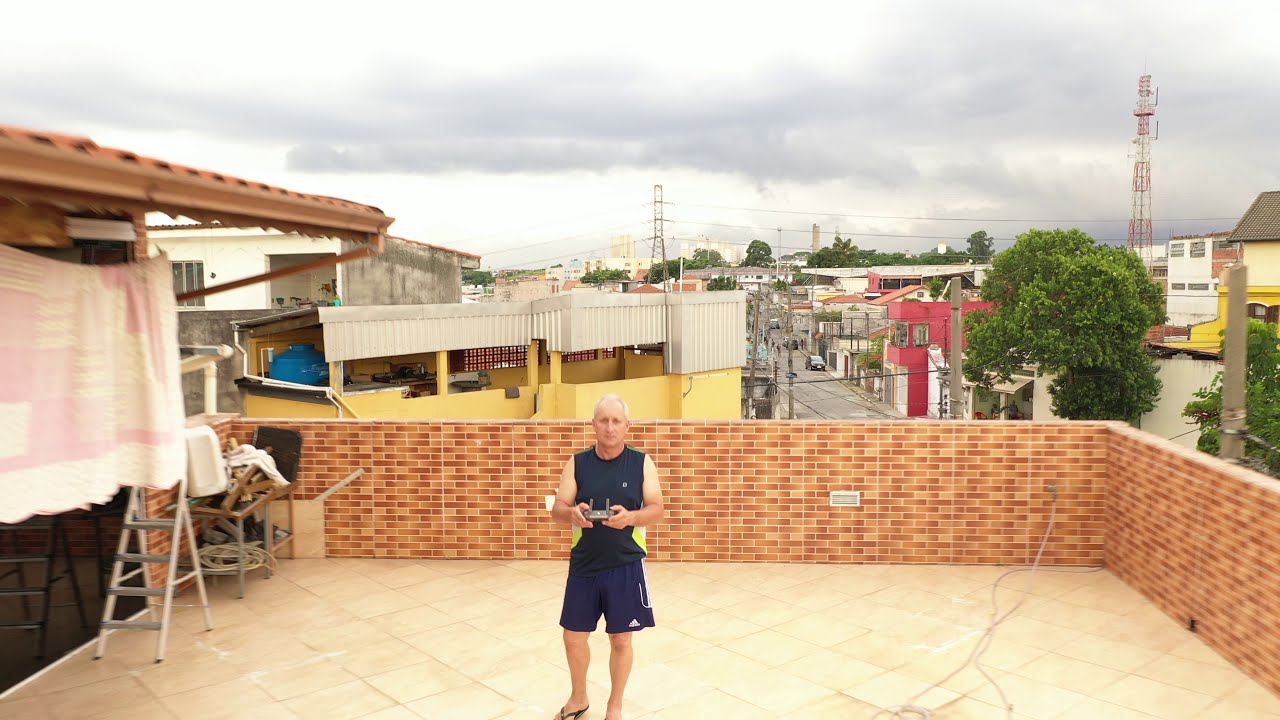In a slightly run-down urban area, a bald man in his 40s to 60s stands on a yellow-tiled rooftop terrace surrounded by a brick wall. He is wearing a blue sleeveless shirt, navy blue shorts, and flip-flop sandals, and he holds a remote controller, likely for a drone. The foreground reveals a partial roof, a ladder, a pink and white blanket hanging from a clothesline, and some coiled hose under a table. Beyond the rooftop, the background shows a gray, cloudy sky, several nearby buildings including red and yellow ones, utility poles, and a tall tower. The scene portrays an everyday moment amidst a neighborhood of diverse structures and everyday objects.